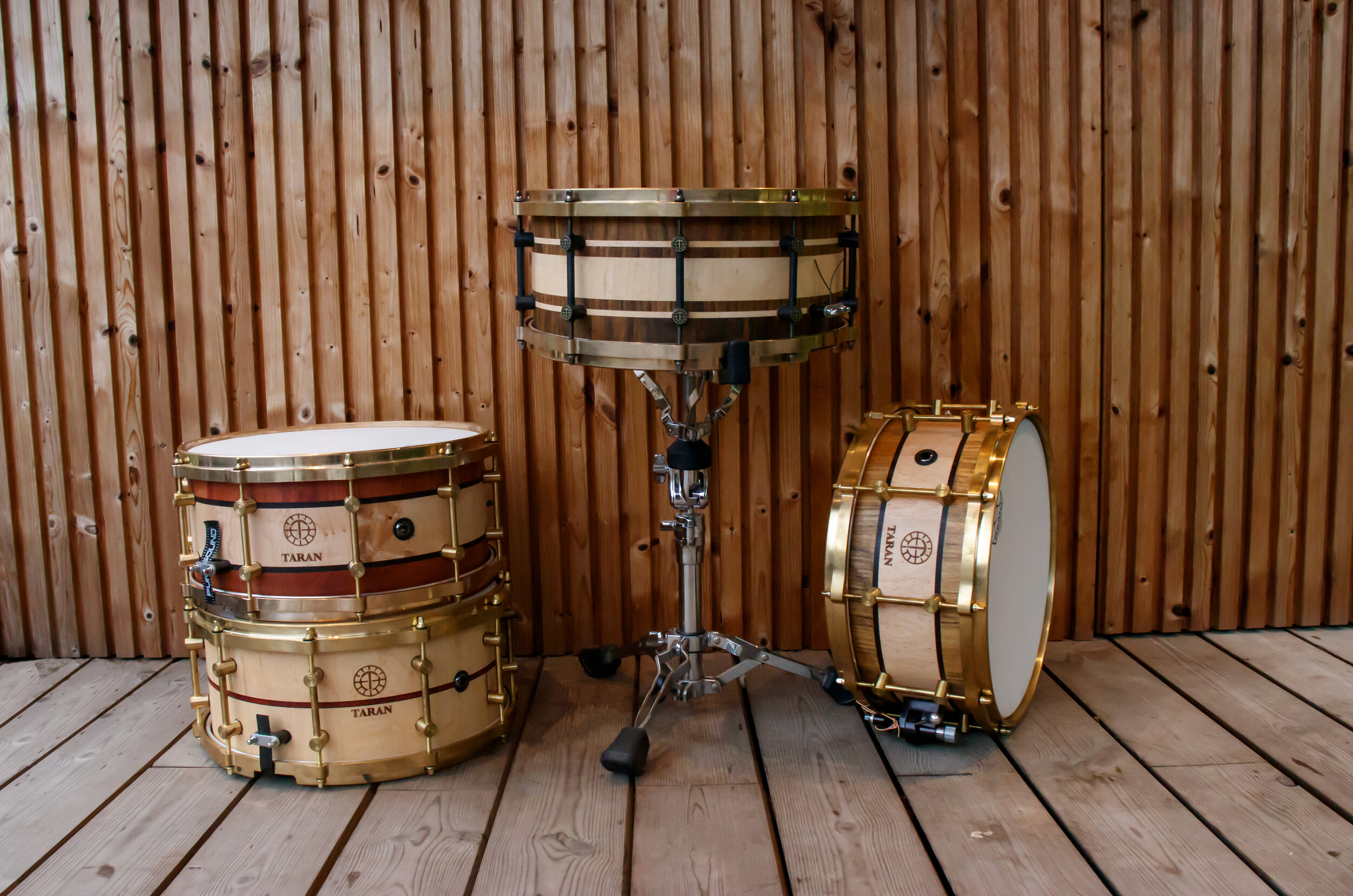The image showcases a collection of four Taran drums arranged on a wooden decking with a slotted wooden fence as the background. The background fence features vertical strips of dark brown wood with visible knots, while the decking is made of lighter-colored wooden planks. On the left side of the image, two round drums are perfectly stacked on top of each other. The top drum has a brownish color with a maroon tint, while the bottom one is more of a cream shade. Positioned in the middle, a drum is mounted on a metallic tripod stand with black padded holders. This drum has a creamy center stripe with a dark wooden outline and a copper-colored rim. To the right, another drum rests on its side with a similar color pattern, featuring gold, brown, and tan hues. Each drum bears the name 'Taran' and shares a consistent design of brown stripes, cream centers, and brass-colored rims.